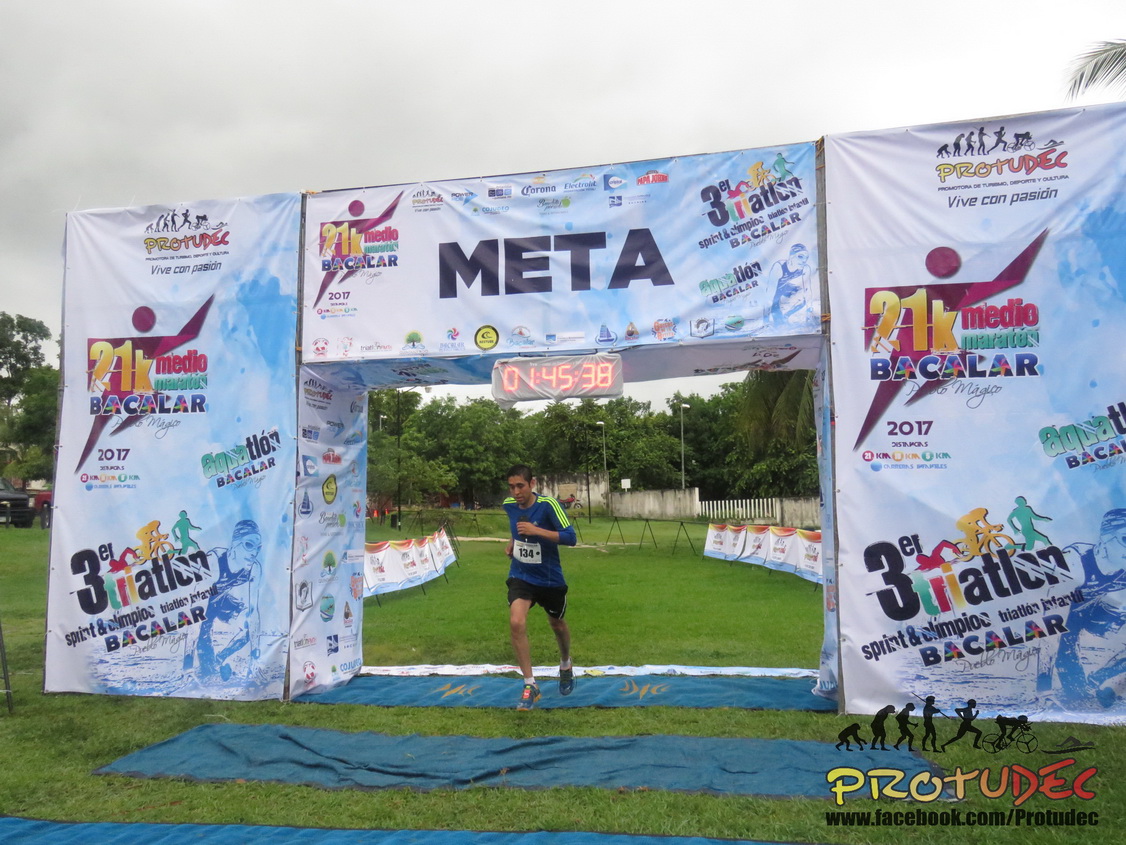The photograph captures an overcast day at the finish line of a race. A man, wearing blue and numbered 134, runs through a large, decorated barricade adorned with various advertisements and sponsor logos. Prominently displayed at the top of the barricade are the words "META 21K Medillo Baccalaureate 2017 3ER Triathlon Spirit and Champion Baccalaureate" in blue letters. The finish time displayed overhead reads 1:45:38. The structure features bluish-white signage accented with purple and green colors, and below it are long blue tarps spread over the grassy ground. In the bottom right corner, the banner shows "Pro2Deck" alongside a Facebook link (www.facebook.com/Pro2Deck). The scene also includes images of a bicyclist and a runner, underscoring the event's triathlon theme. Trees are visible in the background, contributing to the outdoor, natural setting.